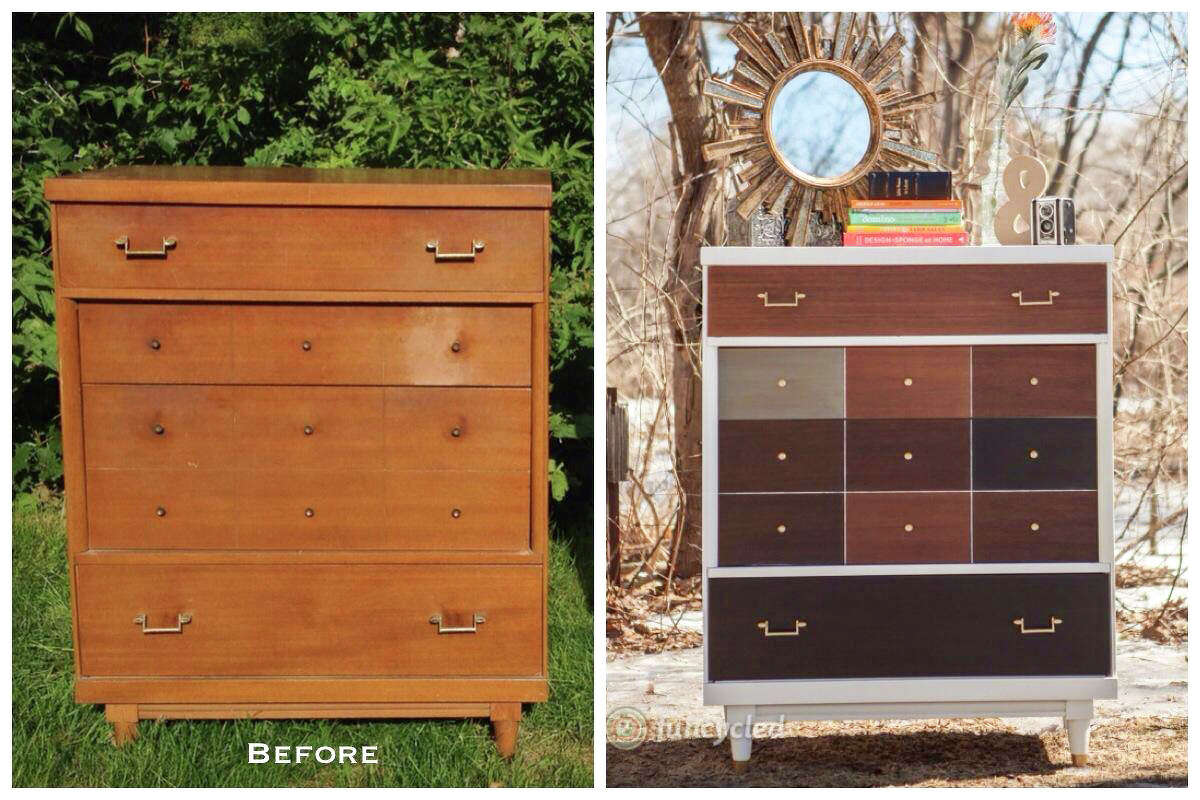The image is a detailed before-and-after transformation of a brown wooden dresser, divided into two equal parts with the "Before" on the left and the "After" on the right, both positioned in outdoor settings.

On the left side, the dresser features a natural honey-brown wood finish, set against a lush background of green grass and vibrant trees. The dresser has a top drawer with two handles, one on each side, followed by a piece of wood that extends horizontally below it. There are three rows of drawers beneath this piece, each equipped with three knobs, and a bottom drawer mirroring the top with two handles. 

The right side showcases the same dresser, but with a significant makeover. Now outlined in white, the dresser's top drawer sports a darker wood, while the nine knobs on the middle drawers boast a variety of colors: gray, light brown, dark brown, and black. The bottom drawer is a solid black with white legs supporting it. Atop the dresser sits a small stack of items, possibly books, and what appears to be a cup on the right. Above it, a decorative element resembling a round wooden circle with radiating projections hangs. The background contrasts with mostly bare trees and sandy ground, indicating a change in season or location.